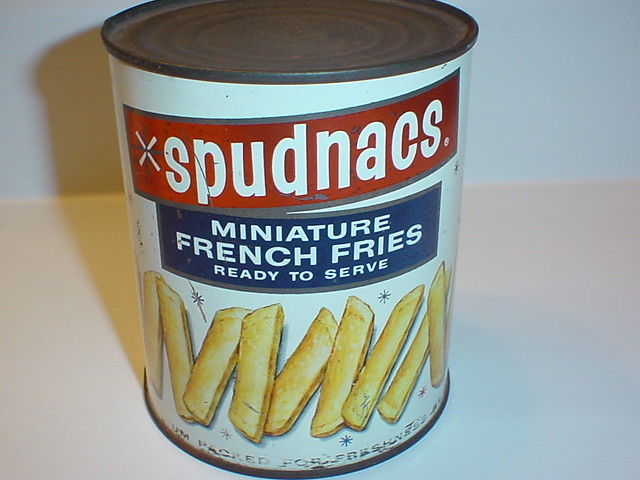The image depicts a vintage can of miniature French fries, likely from the 1960s or 70s, resting on a white surface that casts a shadow behind it, with a plain white wall as the backdrop. The slightly angled photo cuts off the top of the can but offers a clear view of its faded, somewhat battered appearance, which adds to its old-fashioned charm. The label on the can is predominantly white with a traditional silver tin finish at the top and bottom. The prominently featured brand name "Spudnax" is displayed in whimsical red lettering within a long red rectangle bordered by silver, matching the tin lid. Below it, a blue rectangle with a matching silver border announces in bold white capital letters "MINIATURE FRENCH FRIES," followed by "READY TO SERVE" in smaller text. The central graphic showcases a colorful illustration of thick-cut potato wedges, rendered in pale and mustard yellow hues. At the bottom of the label, though partially illegible due to wear, the word "packed" is visible near the left-center, accompanied by star-like asterisks. The retro design and aged condition of the can suggest a nostalgic artifact from a bygone era.